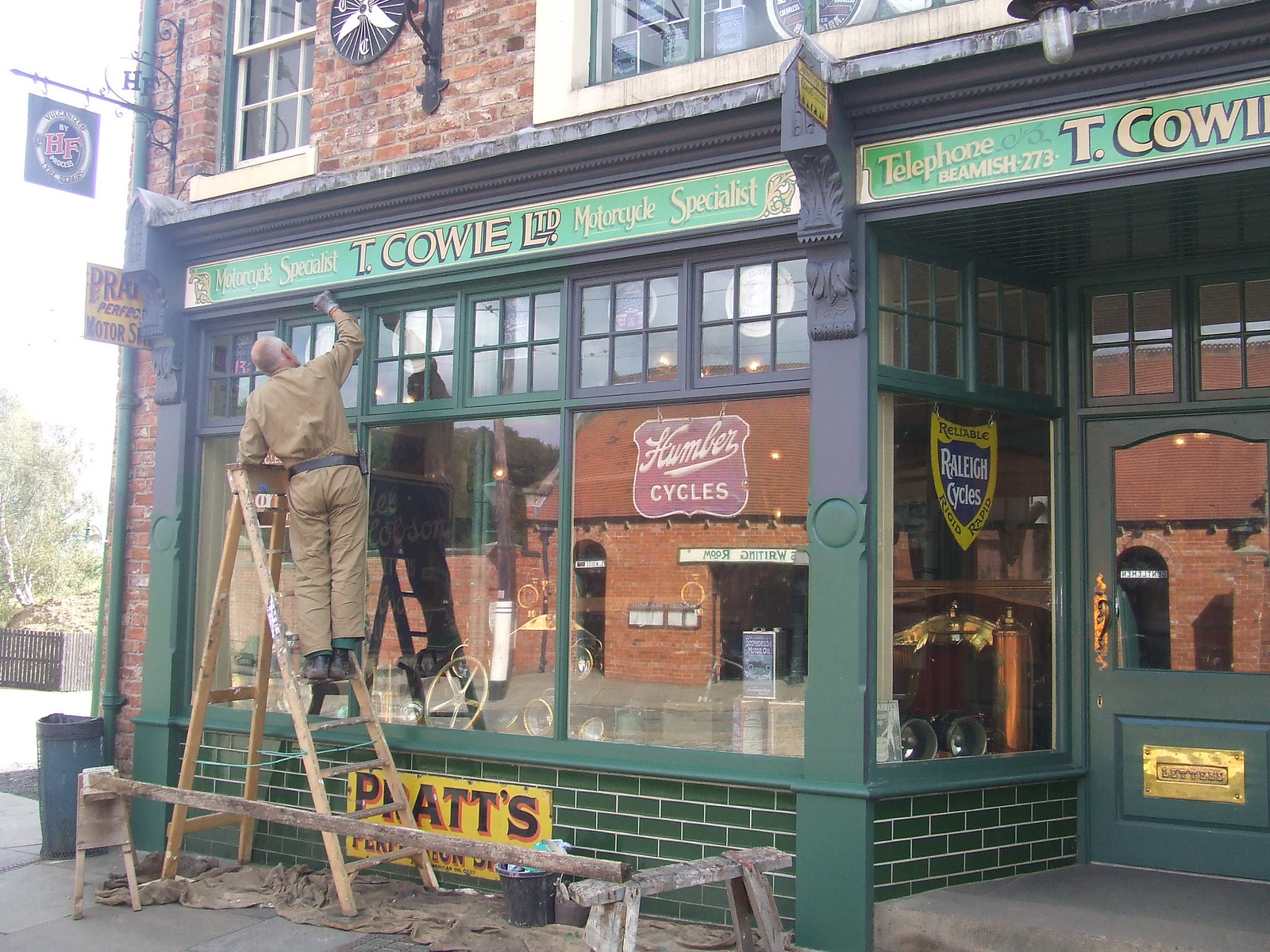The image depicts the exterior of a small brick pub adorned with green accents and numerous paned windows. Central to the scene is a man dressed in a brown uniform—comprising a brown shirt, brown pants, a black belt, and black shoes—working diligently on a stepladder. This man, who is also wearing gloves, appears to be either painting or cleaning the building's trim.

Above him, a green banner with yellowish letters reads "T. Cowie LTD, Motorcycle Specialist, Telephone Beamish 273." The windows below the banner display various signs: one window features a red sign that says "Humber Cycles," while another showcases a yellow sign that reads "Raleigh Cycles." The building's entrance is marked by a green door to the right, and additional signs with placards can be seen near the door and other areas of the façade.

The man is surrounded by equipment, including a tarp, a dirty rug, and buckets, all visible below the ladder. The layered window arrangement—with smaller window panes above and larger ones below—adds to the charm of this quaint establishment.